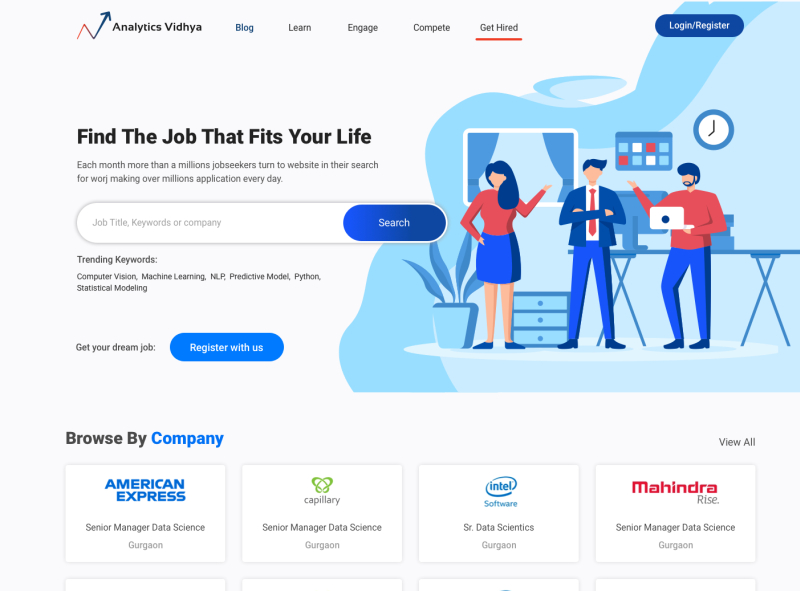The image showcases the homepage of a website called Analytics Vidhya. The header features the logo and name of the website in the top left corner. Alongside this, spanning from left to right, are several headings: 'Blog' highlighted in blue, followed by 'Learn,' 'Engage,' 'Compete,' and finally, 'Get Hired,' with the latter underlined in red. In the top right corner is a blue 'Login/Register' button.

Beneath these headings on the left side, large text boldly announces, "Find the job that fits your life." This is accompanied by a brief explanatory paragraph, detailing how users can search for jobs using titles, keywords, or company names. To facilitate this, a search dialog is provided where users can input their desired job title, complete with a blue 'Search' button at the end of the field. Additionally, trending keywords are listed for convenience.

Below this, a prominent blue button encourages users to "Register with us" to help secure their dream job. Adjacent to this text, on the right side of the image, is a cartoon illustration depicting three people standing in an office environment.

At the bottom of the image, an invitation to "Browse by Company" is presented, with 'Company' highlighted in blue. Below this, four white tiles display logos of featured companies: American Express, Capillary, Intel Software, and Mahindra Rise.